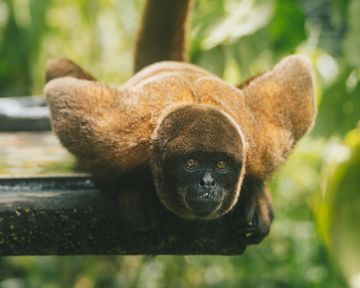This captivating image features a unique monkey, poised on a wooden platform that juts out from the left side of the photo. The scene is relatively dark on the left, with the wooden platform providing the primary perch for the monkey, who is centered in the image. The monkey, with its body hunched down on all fours, appears to be laying flat against the platform, giving a sense of alertness and readiness, almost as if it's prepared to jump onto its prey.

The monkey’s fur is predominantly light brown, transitioning to a darker brown on its head, and its face is entirely black. Its eyes, which are wide open and light brown or yellowish, convey a sense of intensity and alertness. Above its eyes, it has dark brown fur, contrasting with the lighter fur on its shoulders and upper back. One of its black paws is hanging off the edge of the platform, adding to the sense of readiness for action. 

In the background, a tree trunk rises and disappears out of the frame, surrounded by a blur of green, indicating foliage and possibly jungle, creating a natural, lush environment. The monkey’s raised tail and the description indicating short, soft fur add to the details that make this a striking and engaging portrait of a creature seemingly ready to pounce.